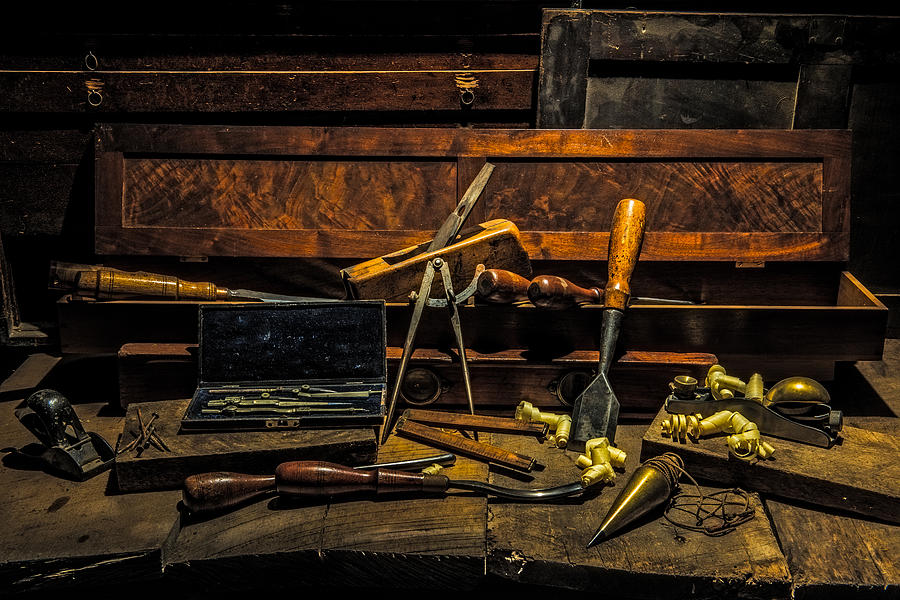The image depicts a dark, vintage-themed workspace featuring a distressed, warped wooden workbench with dark wood tones revealing lighter wood patches. The workbench's surface is cluttered with various hand tools, likely vintage and no longer in regular use. These tools include wood carving and wood shaving tools, scrapers, rulers, and blackened steel implements with old wooden handles in good condition, some featuring red or yellow tones. A string with hooks stretches across the back of the workbench, potentially for hanging additional tools. To the rear of the workbench, two drawers are open, suggesting a toolbox format, and contain more tools along with an object resembling a black cabinet door protruding from one. Scattered on and around the workbench are wooden boxes, including one that is open with a blue velvet liner, displaying various bits and maybe rusted nails. Additionally, an old weight on a string, possibly for marking points, is present among the haphazardly displayed tools. The background is dark, highlighting the contrast between the aged, rugged tools and their refined wooden storage solutions.